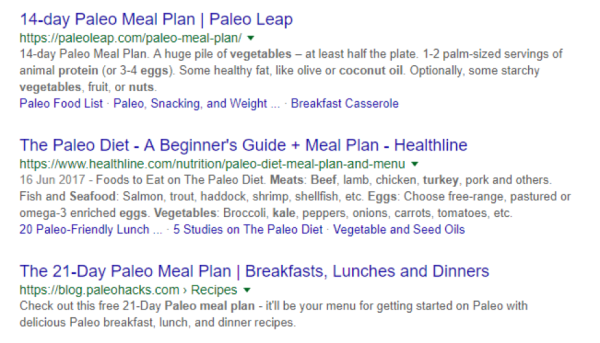The image depicts a Google search results page where someone has likely queried either "Paleo diet" or "Paleo meal plan." Three primary search results are visible, each from different websites. The first result is a "Fourteen-day Paleo meal plan" from Paleoleap (paleoleap.com). The second result is titled "Paleo diet: A beginner's guide, plus meal plan," available on Healthline (healthline.com). The third result, from Paleohacks (paleohacks.com), offers a "21-day Paleo meal plan: breakfast, lunch, and dinner."

Each of these results provides an overview of the Paleo diet, which is based on eating patterns presumed to resemble those of ancient humans, focusing primarily on meats, fats, and proteins. The top two links also have additional sub-pages. The first link includes resources such as a Paleo food list and a recipe for a breakfast casserole, while the second link features five studies on the Paleo diet along with discussions on vegetable and seed oils. This suggests that the diet encourages the consumption of natural, unprocessed foods and excludes common modern dietary components like grains and processed sugars.